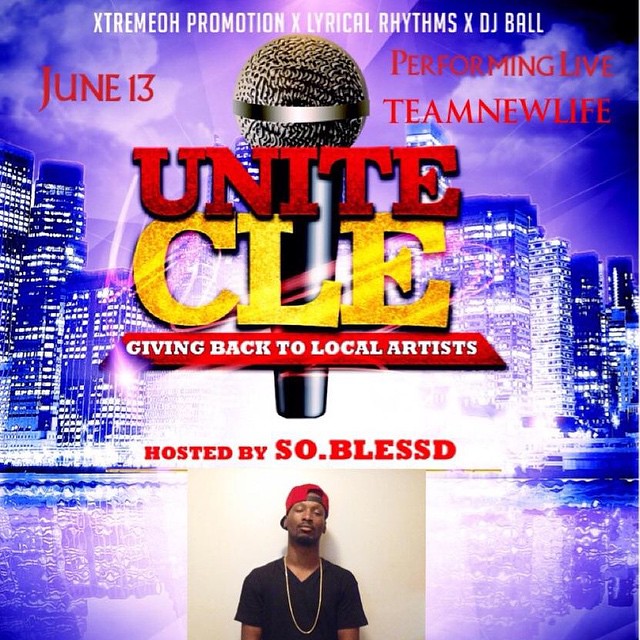The promotional flyer features a vibrant cityscape background tinted in purple and blue hues, set alight with energy streaks and lens flares. Dominating the center of the image is a large, superimposed photograph of a microphone. Just above, the headline in bold white text reads "ExtremeO Promotion X Lyrical Rhythms X DJ Ball," clearly marking it as an event advertisement. The word "Unite" appears in large red letters followed by "CLE" in gold, emphasizing Cleveland, with a tagline in white that says "Giving Back to Local Artists."

To the left of the microphone, red text announces the event date: June 13th, while on the right, similar red text promotes the live performance by Team New Life. At the bottom of the flyer, the red text "Hosted by So Blessed" draws attention to the host, whose image is also featured. The host is a black man sporting a black t-shirt, a backward red baseball cap, and a gold chain. The image remarkably blends detailed elements with striking colors to capture attention and provide all necessary event information.